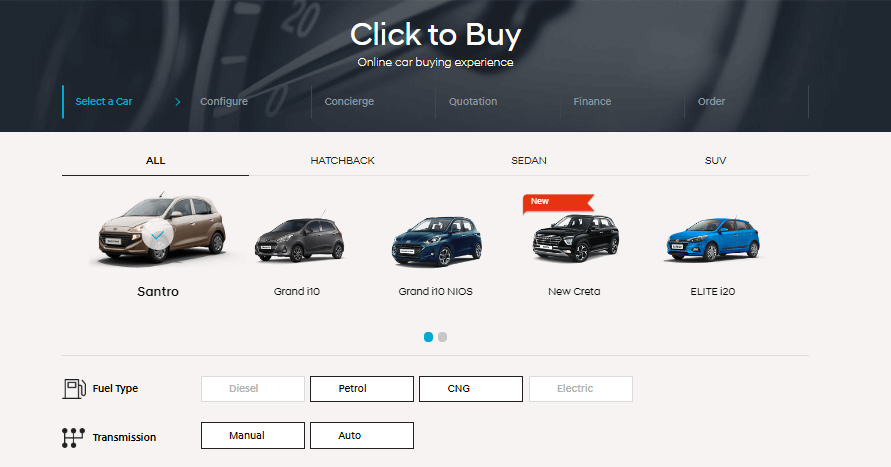A screenshot of an online car-buying website interface, primarily displayed in landscape orientation, wider than it is tall. At the top of the page, a solid black banner spans the width of the screen. Centered within the banner, "Click to Buy" is prominently displayed in white text, with "Online Car Buying Experience" in smaller font just below it. 

Beneath this, still within the black banner, there are six navigational tabs with faint text. The tab on the far right has a blue underline and is highlighted in blue, indicating it is selected; the tabs might include categories such as "Configure," "Questions," "Finance," and "Order."

Below the black banner, the background transitions to gray, where car selection options are displayed. Four tabs labeled "All," "Hatchback," "Sedan," and "SUV" sit at the top of this section. The "All" tab is highlighted with a black underline. 

Centered below these tabs are images of five different cars with corresponding model names underneath. The model on the far left is a "Santro" and is slightly larger than the others, marked with a green checkbox indicating selection. The fourth car over features a red banner that reads "New."

Beneath the car images are navigation buttons, a blue button and a gray button, indicating that the user is on page 1 of 2. 

At the bottom, a thin gray line spans the width of the screen. Below this line, filter options are available. On the left, there are four fuel type options displayed as square icons labeled "Diesel," "Petrol," "CNG," and "Electric," with "Petrol" and "CNG" selected. On the right, transmission options are shown, with icons for "Manual" and "Auto," and both options are selected.